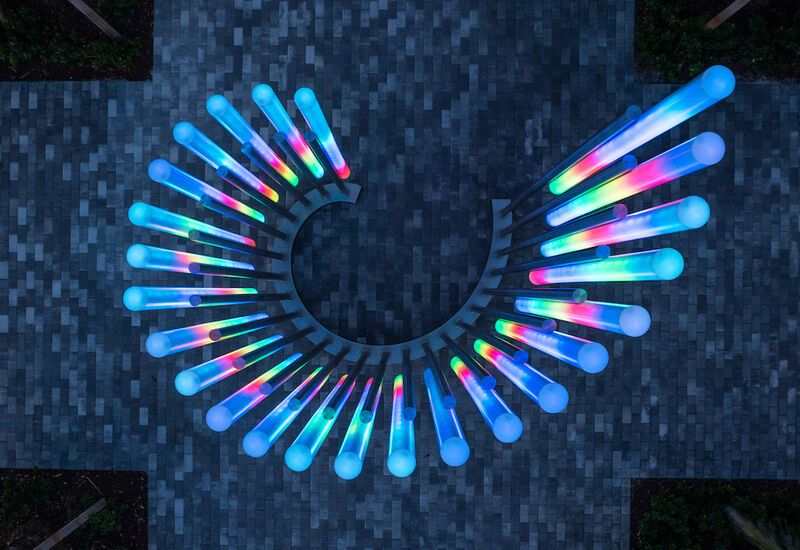This image depicts a digitally rendered, CGI-like scene viewed from a top-down perspective, showcasing a complex, almost optical illusion-type structure. This structure consists of around 20 to 30 long blue cylinders, which transition into a rainbow of colors—red, yellow, and green—along their length. The cylinders appear to be illuminated from within and are mounted on metal rods, forming an asymmetrical, horseshoe-shaped arrangement. The photograph seems to have been taken in a dimly lit environment, possibly a museum exhibit, emphasizing the vibrant glow of the cylinders against the darker backdrop. The scene is set against a floor composed of bluish tiles, featuring a mix of blue, black, white, and gray hues. Additionally, four potted plants are strategically placed in each corner of the scene.